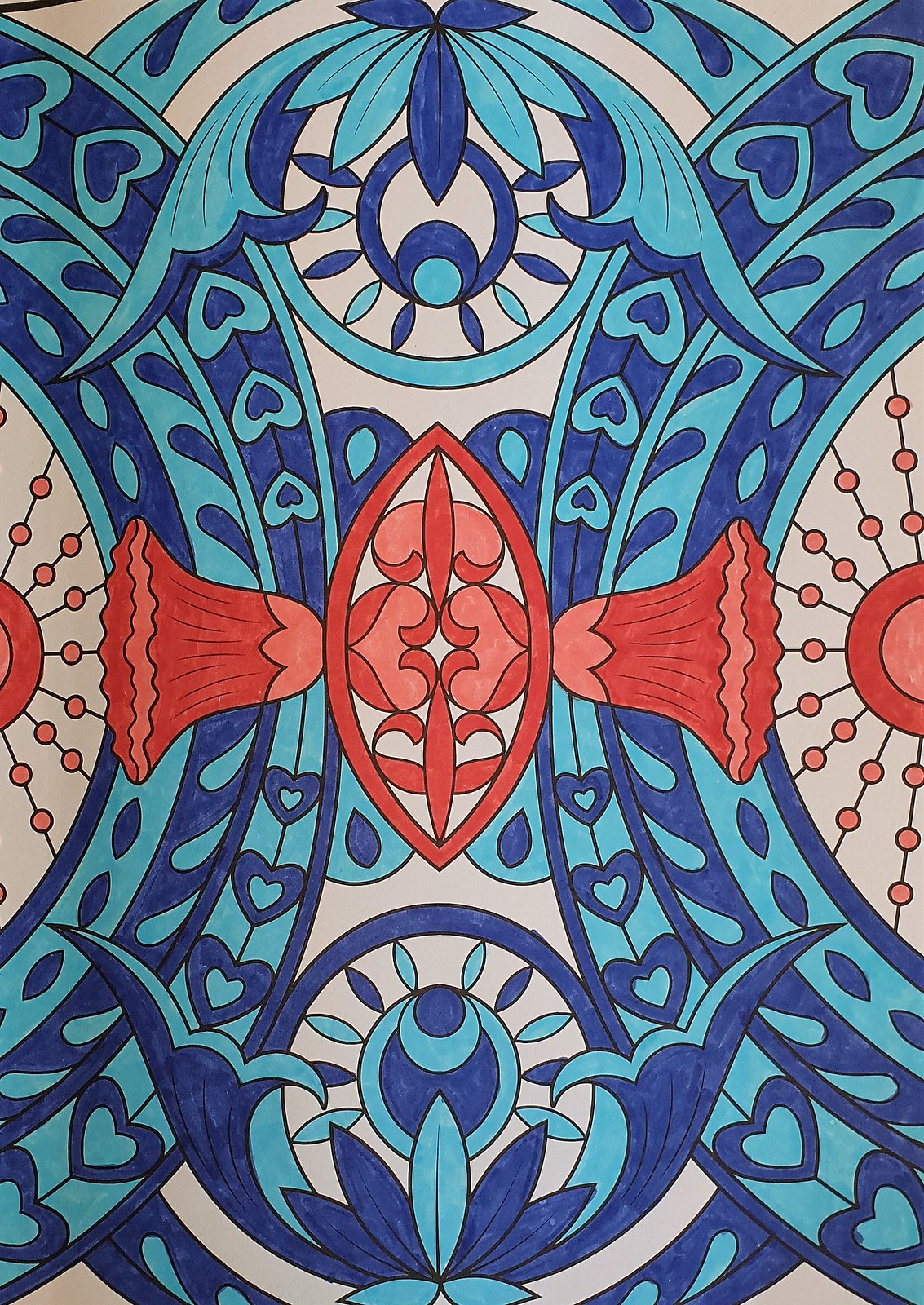The image is a detailed and intricate floral design rendered in an array of royal blue, light blue, darker pink, lighter pink, dark red, light red, and touches of cream. The overall pattern is reminiscent of old-fashioned wallpaper typically found in historical homes or churches. The design features symmetrical, mirrored elements with each side reflecting the other. The central motif consists of tulip-like, bell-shaped flowers surrounded by swirling blue flower shapes and ribbons, interspersed with small hearts and beaded accents. The pattern also includes teardrop shapes, leaves, petals, and circles, creating a psychedelic yet elegant look, akin to the intricate designs found on Turkish ceramics or vintage pottery. The floral and geometric elements are arranged in a manner that suggests the design could be used as a decorative piece, perhaps in a Wayne's coat style along a stairway, enhancing the vintage charm.